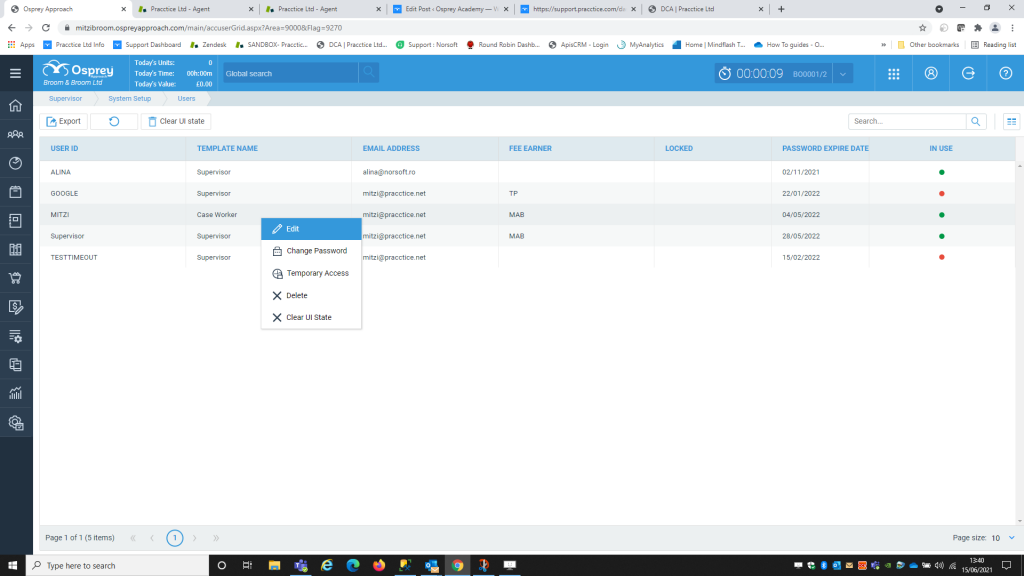The image is a detailed screenshot of a computer interface for the Osprey Approach software. In the top-left corner of the screen, the text "Osprey Approach" is prominently displayed. Below this, there is an address bar, underneath which a sidebar features several options, including "Apps," "Practice," "Limited Info," "Support Dashboard," "Zendesk," "Sandbox Practice," and "DCA Practice," among others. The sidebar has a black background and includes icons such as a house, a clock, a folder, a shopping cart, and a gear with a question mark next to it.

A blue banner runs horizontally across the screen with the text "Osprey, Broom and Broom Limited." Below the banner, there are tabs labeled "Supervisors," "System Setup," and "Users." This section also has buttons labeled "Export," a circular arrow for resetting states, and a button that says "Clear UI State."

The main content area is divided into seven columns, each with blue headers. The column headers are "User ID," "Template Name," "Email Address," "Fee Earner," "Locked," "Password," "Expired Date," and "In Use." Listed under "User ID" are values such as "Alina," "Google," and "Test Timeout."

Floating above this grid is a rectangular box with the word "Edit" at the top. Below it are four buttons: "Change Password," "Temporary Access," "Delete," and another "Clear UI State."